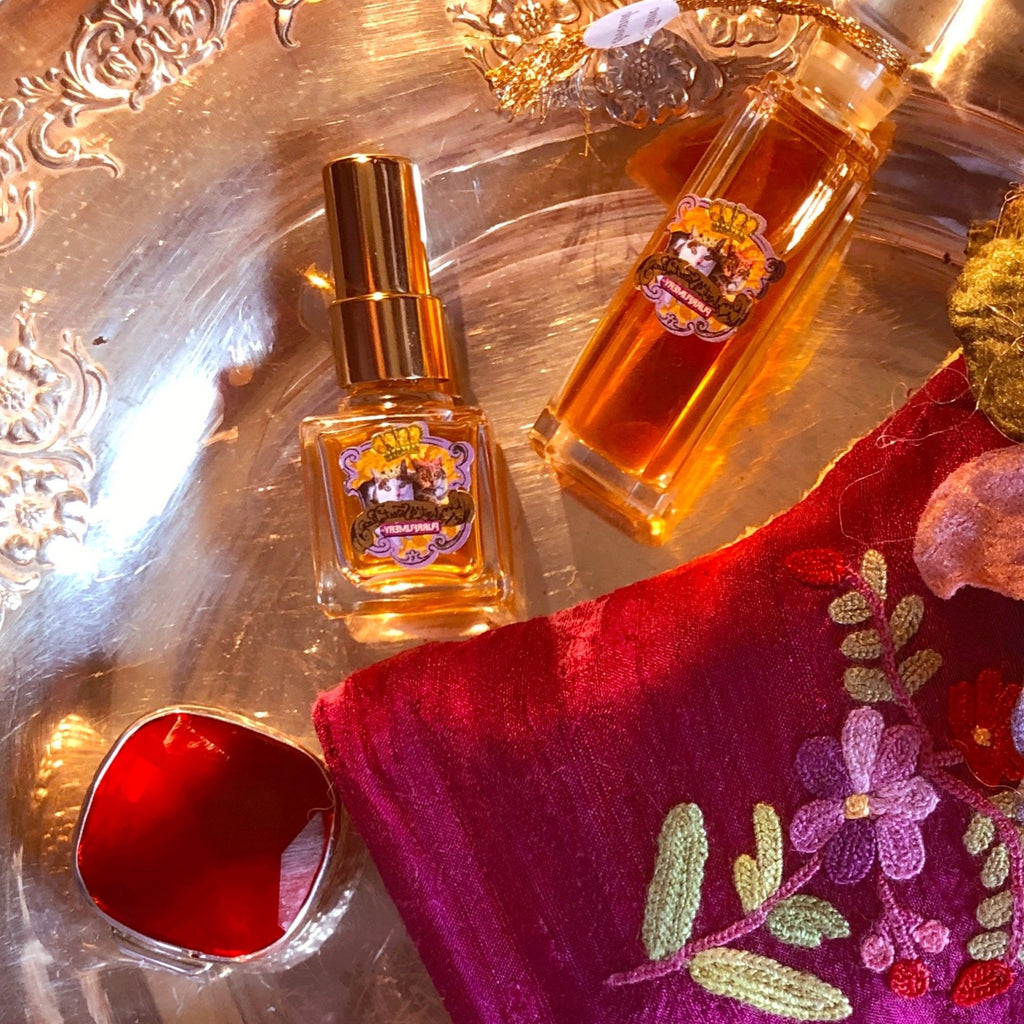This photo captures a detailed and vibrant still-life arrangement. At the center, a glass plate features a striking red cloth adorned with a meticulously crocheted design. The crocheted motif includes a prominent stem with pairs of verdant leaves on either side, culminating in a bouquet of multi-colored petals displaying various shades of purple. Scattered amongst these are smaller red flowers, adding pops of color to the composition. In the upper right corner, a bowl filled with lush green moss adds a touch of natural texture. Two elegant containers, one possibly a perfume bottle and the other a lipstick tube, accompany the scene. The lipstick tube displays a pale brown hue, while a striking red and silver container holds a dark red substance, adding an air of mystery. The entire arrangement rests atop a wooden table, the natural grain of the wood visible beneath the glass plate, grounding the vivid and eclectic display in an organic setting.